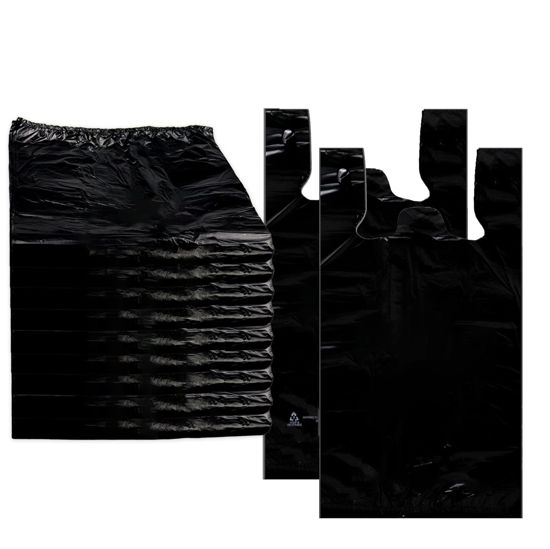The black and white photograph features a prominently large stack of black t-shirt style plastic carry-out bags on the left side. These bags are commonly seen in corner stores or hair stores and are relatively small compared to typical grocery store bags. Two of the bags are displayed upright on the right side, clearly showing their t-shirt handles and central tab for hanging on store hooks. One bag has a white recycling symbol printed on it. The bags appear on a white background, which emphasizes the contrast and details, suggesting that this might be a product information photo from a catalog or an online source for restaurant supplies.